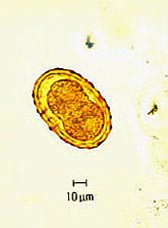The image is a vertical rectangle, approximately one and a half times as tall as it is wide, with an ivory or off-white background, resembling stained white. Centrally positioned at the bottom, there is a scale marked "10 µm" (micrometers) in gray or black text, with a horizontal line flanked by two vertical bars. The focal point of the image is an oval-shaped cell, oriented upwards and slightly to the left. The cell features a speckled brown interior and is bordered by a yellowish outline. Additionally, on the right side, there are green dots and smudges scattered around. The image appears to be a detailed microscopic view of a cell, capturing its intricate structure and scale.